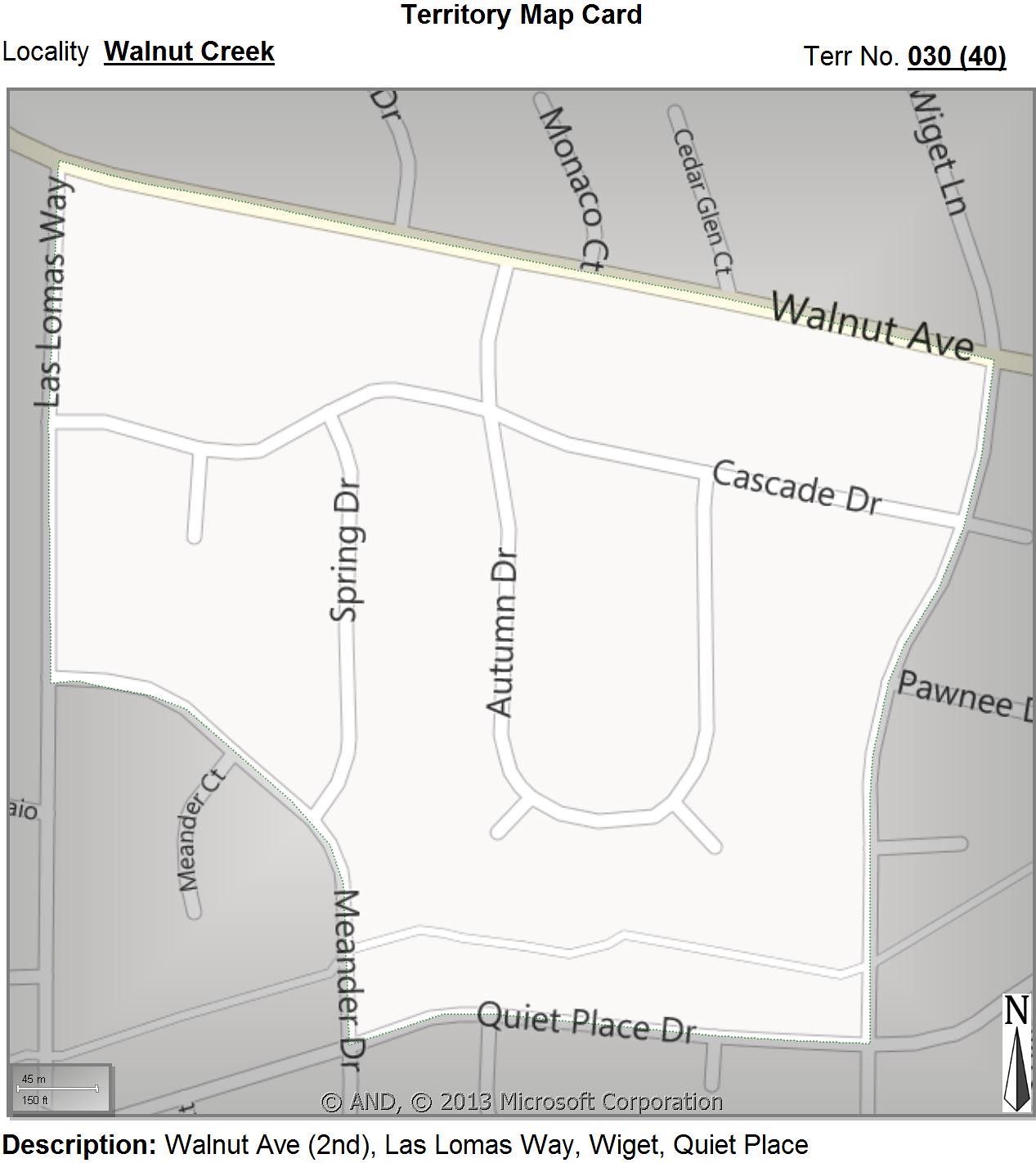The image is a screenshot of a map, likely sourced from Google Maps or a similar digital mapping service, showcasing a specific area of Walnut Creek. At the top of the image, there is a title in black text that reads "Territory Map Card." In the top left corner, "Locality: Walnut Creek" is displayed prominently in dark black text with an underline. The top right corner of the image features additional text: "Terr. No.: 030 (40)" in the same dark black text.

The map itself highlights a particular section with a white glow surrounding specific streets, while the areas outside this glow are darkened, emphasizing the designated territory. Within this highlighted portion, several streets are clearly identified: Walnut Avenue, Las Lomas Way, Quiet Place Drive, and Meander Drive. Other streets within the bright section include Autumn Drive, Spring Drive, and Cascade Drive.

At the bottom of the image, there is a description that lists key streets in the highlighted area: "Walnut Avenue, Las Lomas Way, Widget, Quiet Place."